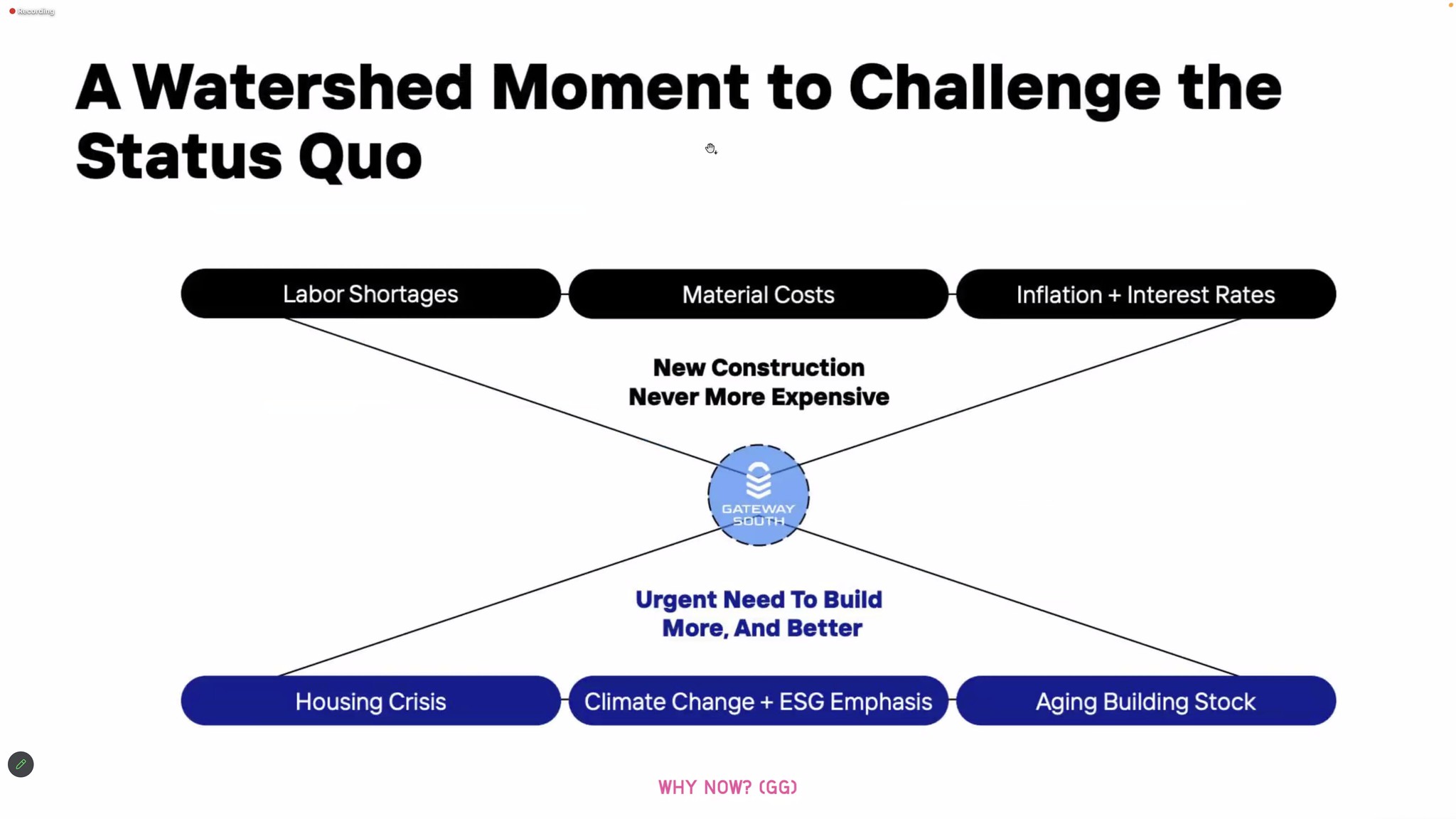The image, likely part of a presentation, showcases a detailed diagram under the prominent title in large black font, "A Watershed Moment to Challenge the Status Quo." Below the title are three horizontally arranged black bars, each containing phrases: "Labor Shortages," "Material Costs," and "Inflation Plus Interest Rates." Under these bars, the text reads, "New Construction, Never More Expensive." Centrally positioned is a blue circle labeled "Gateway South," with lines extending to "Labor Shortages" and "Inflation Plus Interest Rates." Further down, in blue font, it states, "Urgent Need to Build More and Better." The lower part of the diagram features three equally sized purple-blue bars with white text: "Housing Crisis," "Climate Change Plus ESG Emphasis," and "Aging Building Stock." At the very bottom, red letters spell out "Why Now," followed by "GG" in parentheses.